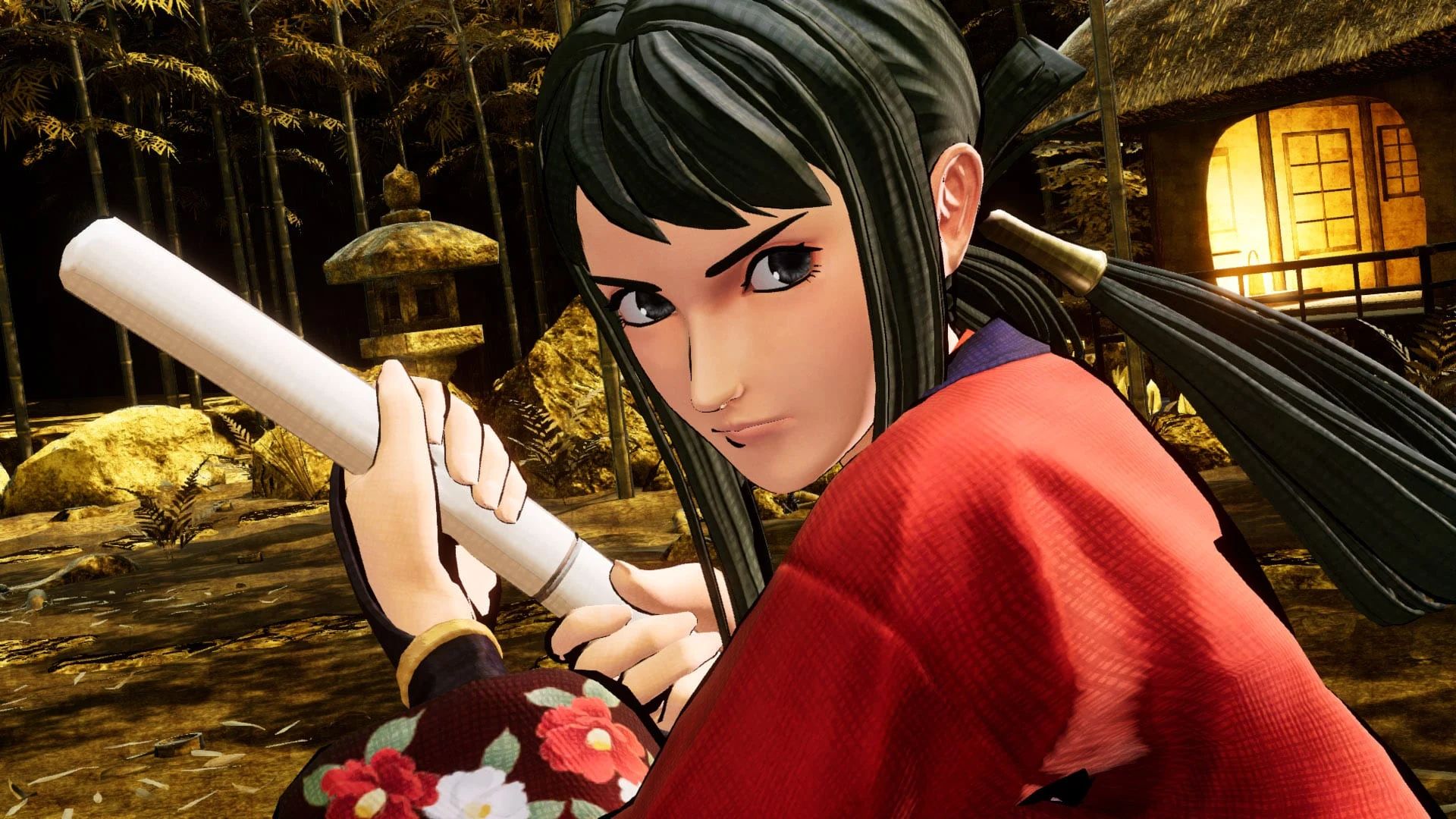The image depicts a three-dimensional, anime-style female character with long black hair tied into a black ponytail and possibly adorned with a ribbon. She has a suspicious expression as she gazes toward the right-hand corner, holding a large, white-handled scroll or cylindrical object in both hands. She is dressed in a striking red robe with a blue collar, patterned with floral designs on the left sleeve and possibly brown-edged at the cuffs. Additionally, she wears gloves that are dark brown on top with white undersides.

In the background, there is a Japanese garden featuring a small stone pagoda, rocks, and sparse trees. To the left of the character, a traditional Japanese hut with illuminated interiors is visible, adding to the authentic Asian ambiance. The setting is further enhanced by additional garden elements like poles, shrubbery, and a serene color palette dominated by natural browns and greens.